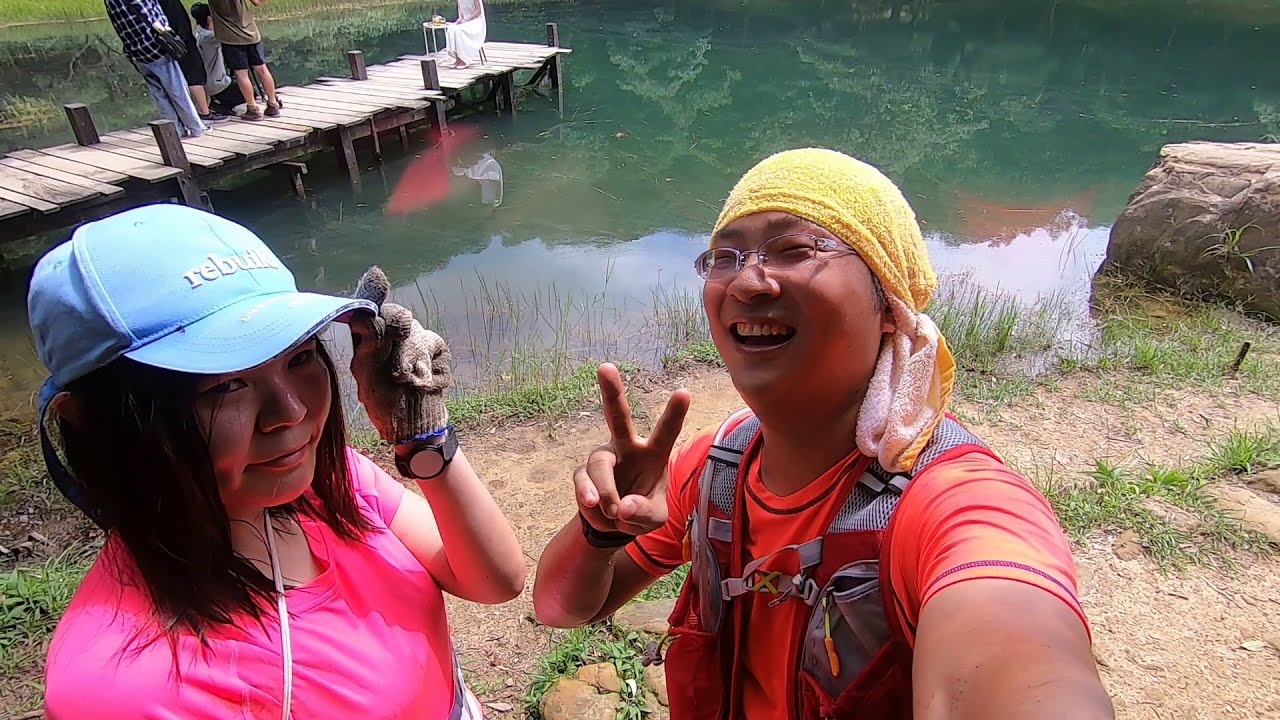In this vibrant outdoor daytime selfie, two young people of Asian descent are positioned in front of a picturesque pond. The man, who is taking the selfie with his arm extended, is sporting thin wire-rimmed glasses and a broad, open-mouthed smile that reveals his teeth. He's wearing an orangish-red short-sleeve shirt paired with what appears to be a gray vest, possibly for hiking or running. A yellow towel is wrapped around his head, styled as a bandana. His right hand is enthusiastically throwing up a peace sign. Beside him to his left, a woman in a pink short-sleeve shirt is captured glancing up at the camera, her blue ball cap with the white text "Rebuild" shading her eyes. She has her left gloved hand lightly touching the brim of her hat, and she's offering a subtle, closed-mouth smile. 

The setting showcases a tranquil pond with bluish-green water reflecting the surrounding forest. The shore is a mix of grass and dusty, rocky terrain. Extending into the pond is a small wooden pier where three or four people are either fishing or chatting, with a chair visible on the pier. The entire scene evokes a serene, outdoor adventure, possibly a hiking trip or a leisurely day by the water.